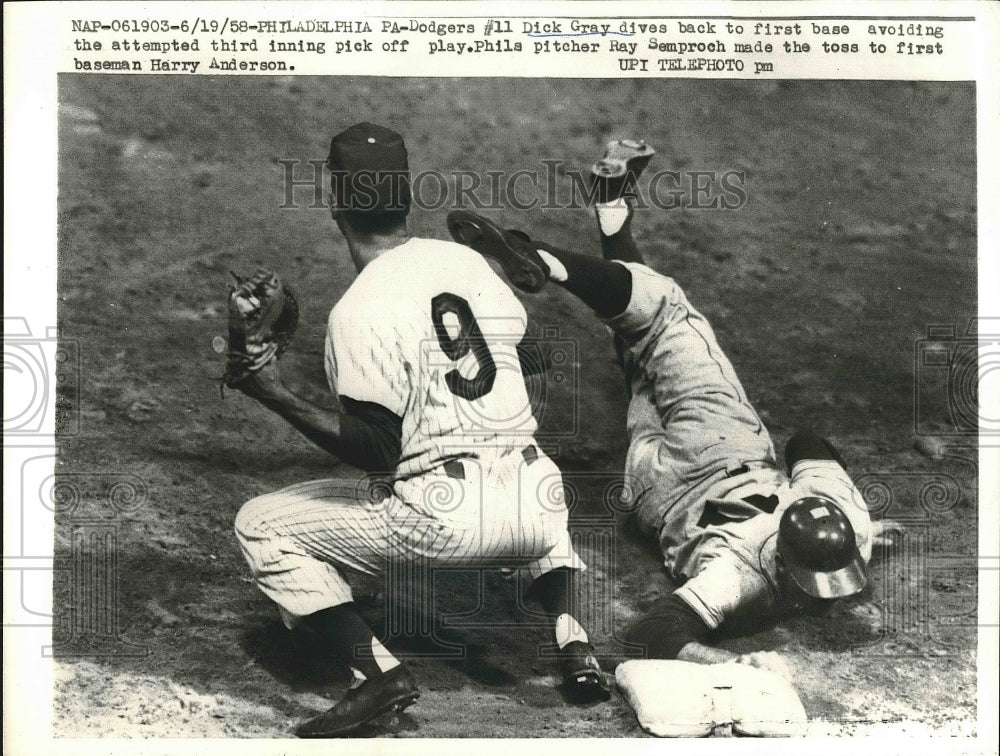This black-and-white newspaper photo captures a dramatic moment in a baseball game. Player number 11, Dick Gray of the Philadelphia P.A. Dodgers, is seen sliding headfirst back to first base, his legs suspended mid-air and dark helmet firmly on. He's attempting to avoid a third-inning pickoff play. His uniform features light-colored short-sleeve shirt and trousers, complemented by dark long sleeves, socks, and shoes. In contrast, the crouching catcher with the number 9 on his back and a catcher's mitt is ready to catch the ball, his uniform featuring a lighter color scheme with dark cap, socks, and shoes. The base stands out as light-colored against the darker field. Above the players, typewritten text identifies the players and play: Dick Gray diving back to first base and Phil's pitcher Ray Semperach making the toss to first baseman Harry Anderson. Watermarks reading "historic images" and repetitive camera graphics streak across the entire image, adding a layer of archival authenticity.